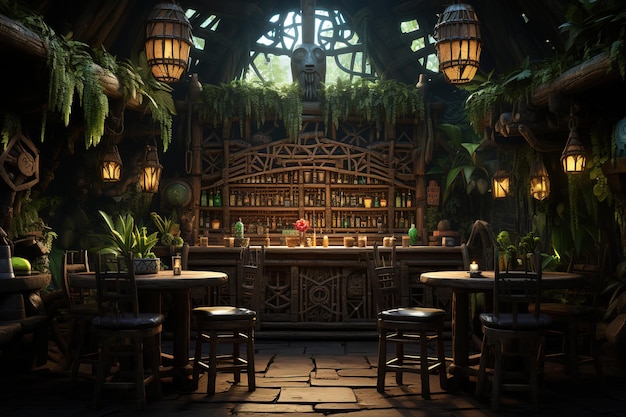This image depicts a detailed, possibly AI-generated or illustrated scene of a forest-themed bar set within a dark, atmospheric building that exudes a fantasy vibe. The centerpiece is a wooden bar situated in the middle, backed by an array of assorted bottles. Surrounding the bar are several brown wooden tables and chairs, each adorned with candles, lending an intimate feel to the environment.

Lanterns of varying lengths hang from the ceiling, providing a warm, ambient light, while greenery and moss drape from wooden beams and walls, enhancing the wild, natural theme. The establishment appears to have skylights, suggested by the light emanating from above, which illuminates the scene despite the overall dark tone of the interior.

A standout feature is the large, mask-like statue with an Amazonian vibe, centrally placed at the back of the image, near the apex of the ceiling, further contributing to the exotic atmosphere. The floor appears rocky, adding to the impression that this bar is an ingeniously crafted outdoor space, seamlessly integrated with its surroundings.